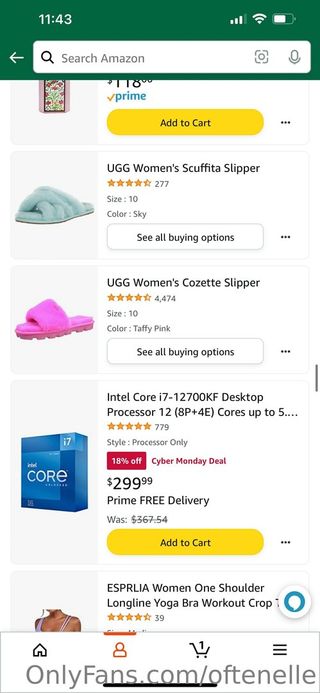This screenshot captures a mobile view of the Amazon app, characterized by its familiar layout. At the top, elements such as the blue "Prime" text with an orange check mark and the "Search Amazon" prompt in the search bar confirm it's Amazon. The phone’s status bar displays the time as 11:43 on the left and a battery meter slightly over halfway full on the right. The top bar, housing the search bar, time, and battery icon, has a dark green background, contrasting with the white backdrop of the rest of the app interface.

Scrolling through the product listings, a mix of women's items and tech products is evident. Partially visible at the very top is a product priced at $118, which includes Prime shipping. The first fully visible product is the "UGG Women's Scuffette Slipper," followed by the "UGG Women's Cozette Slipper," both footwear options. Next is the "Intel Core i7 Desktop Processor," a significant shift from apparel to technology. Concluding the visible section is a "Women's One Shoulder Longline Yoga Bra," showcasing the diverse range of products displayed.